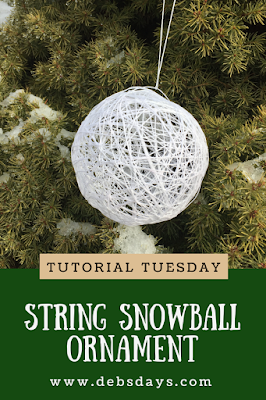The image is an advertisement flyer from www.debsdays.com featuring a tutorial for creating a string snowball ornament. At the center of the image, "Tutorial Tuesday" is prominently displayed in dark text on a green background, with the phrase "string snowball ornament" in white text set against a tan field below it. Beneath these texts, the website www.debsdays.com is also stated in white. The upper part of the flyer showcases a photograph of a Christmas tree still rooted in the ground, lightly covered in ice. A white string snowball ornament is seen dangling from a branch, adding a festive touch to the scene. The image seamlessly combines natural outdoor elements with a crafty holiday decoration, inviting viewers to visit the website for more details.